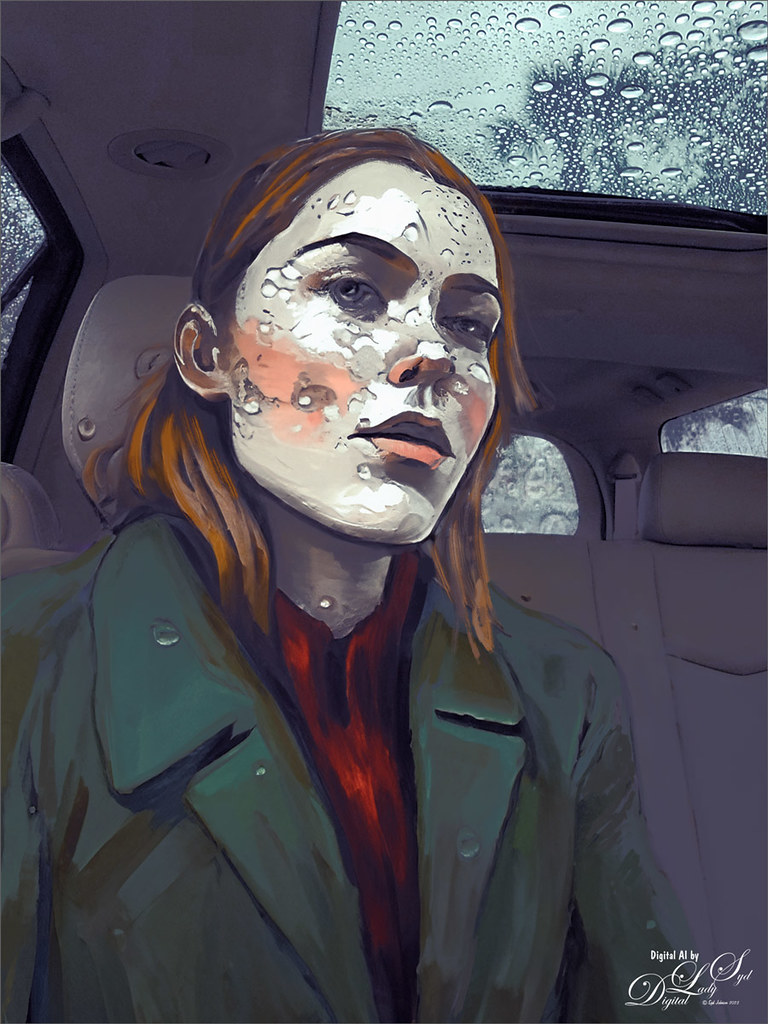This is a digital artwork by Lady Digital, reminiscent of an oil painting. The composition features a blonde woman seated on a grayish bench seat inside a car. She is dressed in a dark trench coat with a large collar, and a vibrant red shirt underneath. Accentuating her features, the woman has orange blush highlighting her cheekbones, nose, and lips. Behind her, a seatbelt is visible on the right, and a portion of the car’s window can be seen, suggesting a backseat view. Adding to the scene is the car’s sunroof, which illuminates the interior with a natural light.